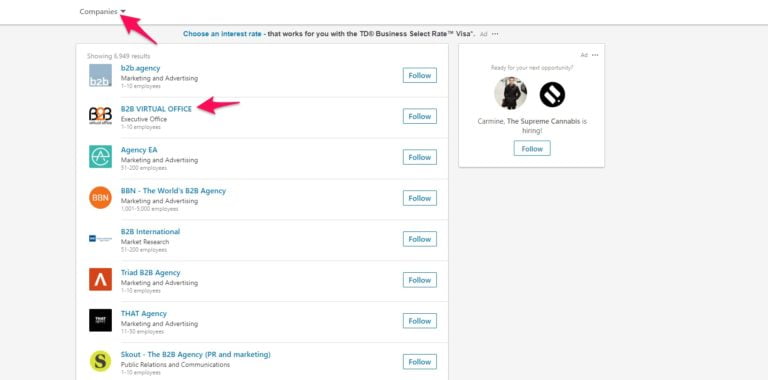The image features a white background with a header at the top that reads "Companies." Below this header, a series of text entries are presented.

1. At the top, there's a purple arrow pointing to the text: "Choose an interest rate that works for you with the TD Business Select Rate Visa."
2. Underneath, several text entries are listed, each representing different business-to-business (B2B) services and agencies:
   - "B2B Agency Marketing and Advertising"
   - "B2B Virtual Office," highlighted with a purple arrow
   - "Agency EA Marketing Advertisement"
   - "BBN: The World's B2B Agency Marketing and Advertising"
   - "B2B International Market Research"
   - "Triad B2B Agency Marketing and Advertising"
   - "That Agency Marketing Advertisement"

At the bottom of the image, there's a gold circle with a black 'S' in the middle. Adjacent to this symbol, the text reads: "AsShout: The B2B Agency PR and Marketing Public Relations and Communications."

The composition is designed to highlight different B2B agencies, focusing on their specialties in marketing, advertising, virtual offices, and public relations. The use of arrows and varying text entries aims to guide the viewer through the options available.